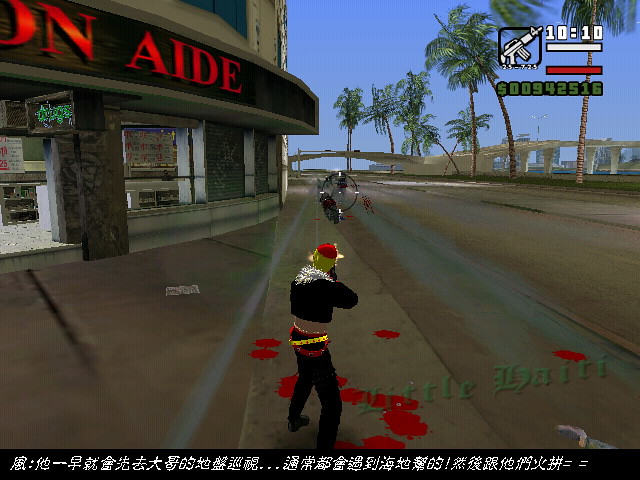This still image, taken from a first-person shooter video game, captures a bustling urban street scene with a distinct East Asian flair. At the very bottom of the frame, a string of Chinese or Japanese characters is displayed, possibly indicating the name of the locale or providing context for the scene. The image depicts a curvaceous building with a marquee, partially visible in the background, marked with the fragmented text "O-N dash A-I-D-E," likely revealing the name of a store or establishment.

Dominating the right side of the screen are several tall palm trees, adding a tropical touch to the otherwise urban environment. Viewed from the perspective of the player character, the focus is on a male figure down the road, who is clearly the target through the scope of a weapon. This target is dressed in black pants, highlighted by a yellow belt, and wears a black shirt and a distinctive red hat.

The composition provides a dynamic blend of urban architecture, tropical elements, and the tense atmosphere typical of a first-person shooter game.